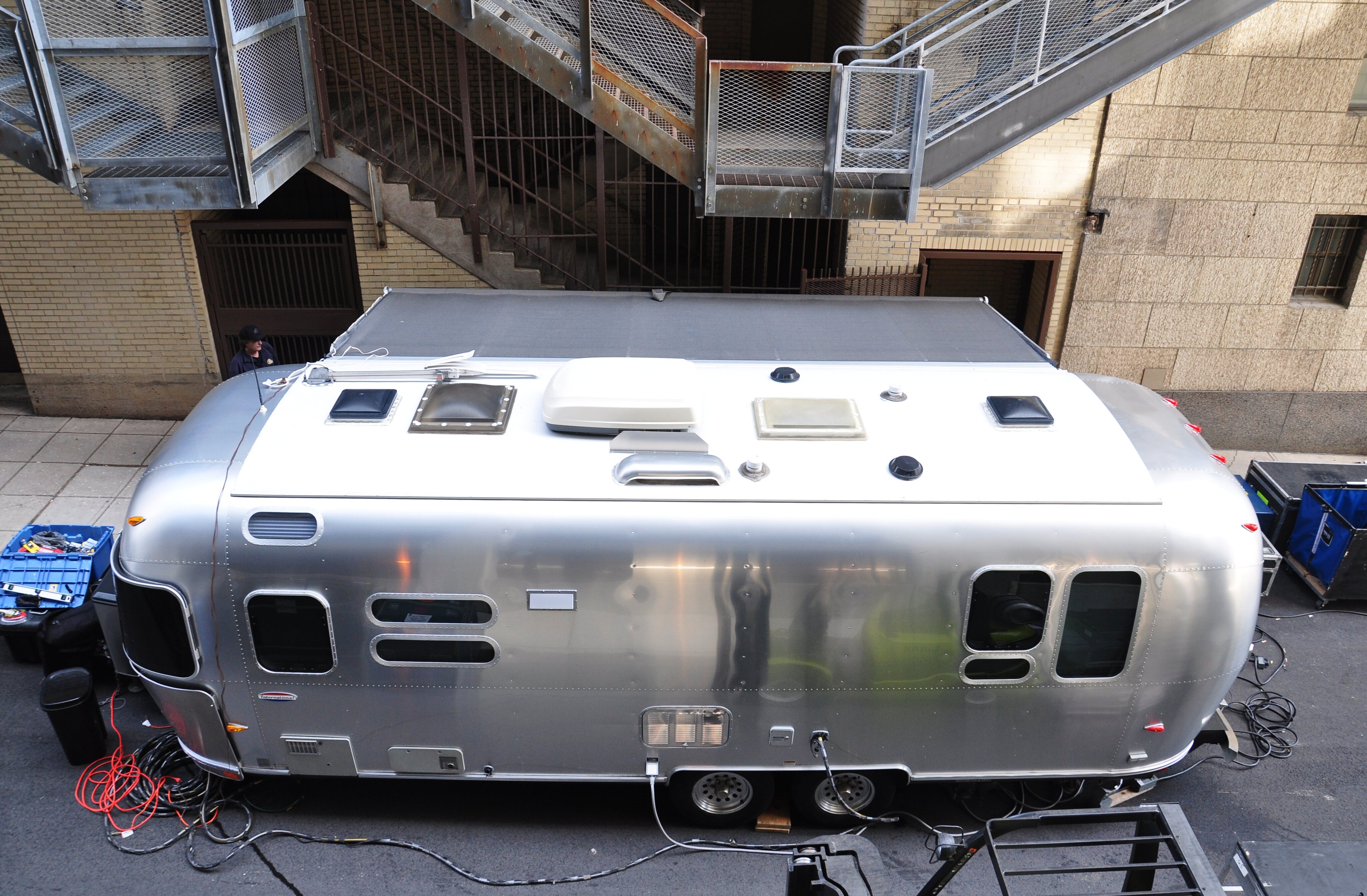The image, taken from an elevated vantage point, showcases a shiny, silver Airstream trailer parked on a relatively empty side street or alley in front of a building. The trailer, possibly being used for filming, has an awning extended and is surrounded by filming equipment, containers, and a plethora of electrical cords plugged into its outlets. Notably, there's an orange extension cord and a black plug on the left side, as well as various other wires and plugs coming out from the front and sides of the trailer. 

Adjacent to the Airstream, there's a security guard standing next to a nearby beige cinder block and brick building that features industrial elements such as metal staircases, multiple levels, and fire exits. The area appears to have some scattered metal boxes and even a garbage can near the trailer. The photograph, taken during the day, shows light reflecting off the trailer, adding a gleaming effect. Despite the urban setting with industrial buildings in the background, the focus remains on the detailed and bustling environment around the Airstream trailer.